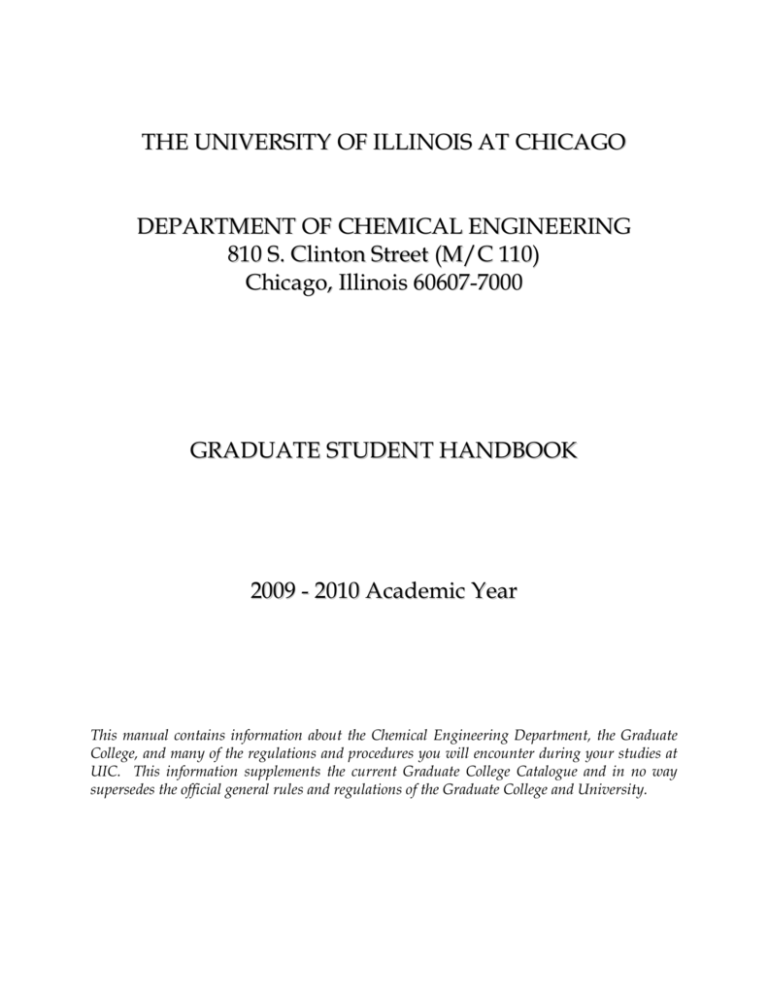Detailed Caption: 

The image features a clean and formal letterhead-style format set against a white background. At the top, prominently displayed in bold black font, are the words "University of Illinois at Chicago". Directly beneath this header, the text "Department of Chemical Engineering, 810 S. Clinton Street (M/C 110), Chicago, Illinois 60607-7000" is shown, also in bold but slightly smaller. Further down, the title "Graduate Student Handbook 2009-2010 Academic Year" is presented in a slightly less bold font, indicating the content's main subject. 

The lower section of the image contains a paragraph in a less bold, gray font, providing detailed information about the handbook's purpose: "This manual contains information about the Chemical Engineering Department, the Graduate College, and many of the regulations and procedures you will encounter during your studies at UIC. This information supplements the current Graduate College catalog and in no way supersedes the official general rules and regulations of the Graduate College and University." 

Overall, the precise and formal arrangement of text effectively communicates the official and informative nature of the document, with distinct typographic hierarchy guiding the reader through the various sections.